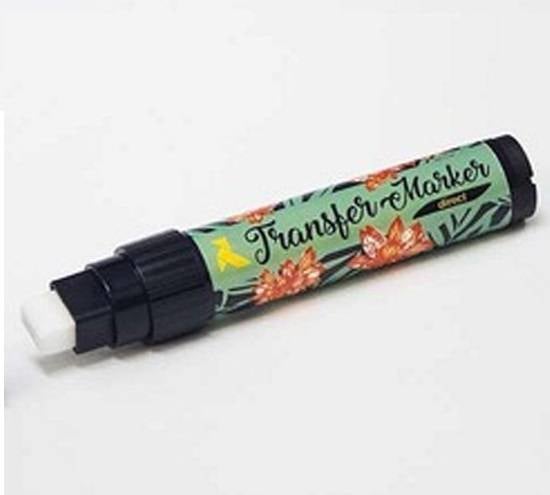In this color photograph, a black plastic marker is laid flat against a pure white background with its white, square-shaped tip on the left. The marker is uncapped, and the cap is missing from the image. A green label wraps around the body of the marker, adorned with a tropical floral design featuring red and orange flowers and dark green palm leaves. Additionally, a yellow object, possibly a bird, is part of the label's intricate design. The label also displays the text "transfer marker" written in cursive black script. Although some details below the "transfer marker" text are illegible due to low resolution and JPEG artifacting, the primary elements and vibrant colors of the marker and its label stand out clearly.